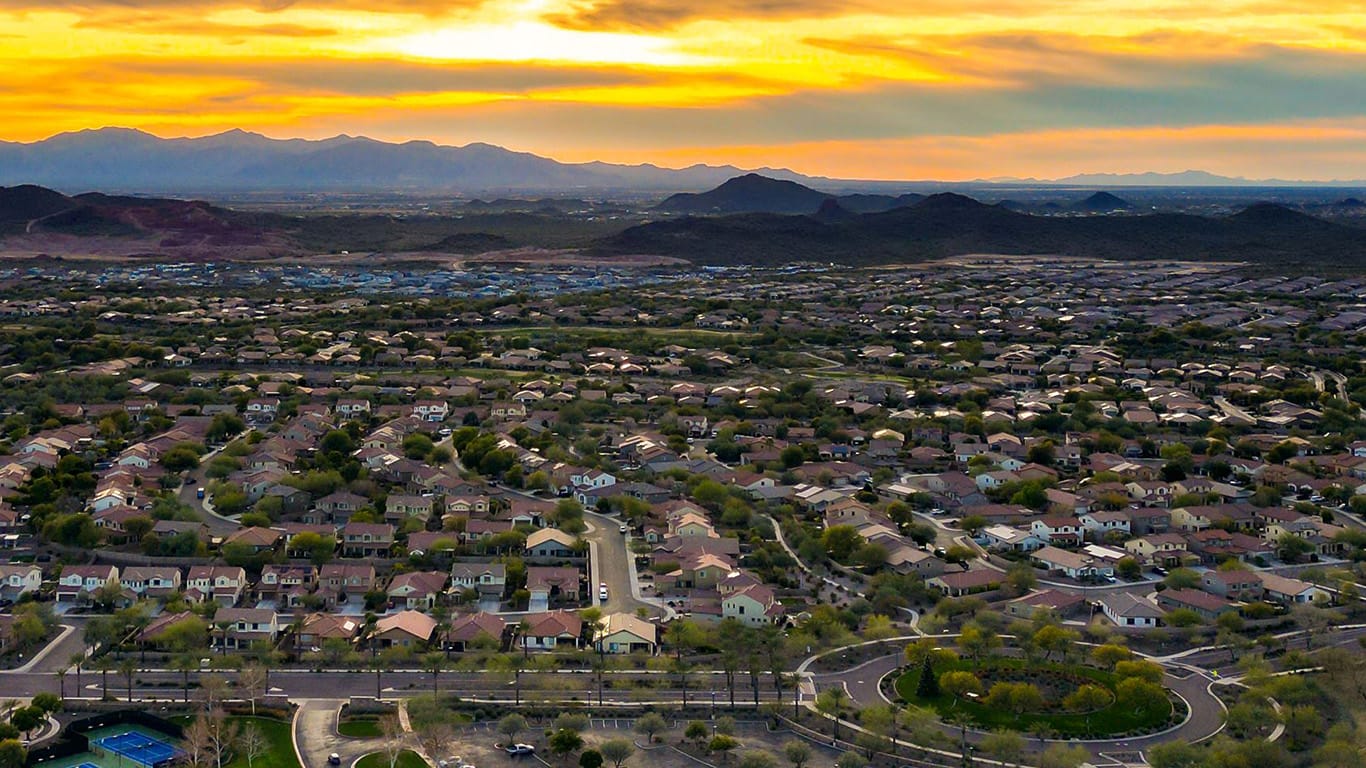This detailed aerial view captures a neatly organized suburban neighborhood at sunset. The bottom half of the image is filled with well-arranged streets and houses, showcasing a diverse palette of roof colors ranging from reds to browns. Trees are abundant, both lining the streets and dotting the landscape, adding to the well-kept impression of the area. A prominent feature in the lower right is a large roundabout, newly paved, with an abundance of trees planted in the center. The main road runs horizontally across the bottom, intersecting with the roundabout.

As the houses stretch up towards the two-thirds mark of the image, they appear smaller and more distant, blending into rows that extend for miles. A mountain range dominates the horizon, its peaks varying in shades of dark grays to blues. In the far background, above the mountains, a breathtaking sunset bathes the sky in vibrant oranges, yellows, and hints of red. The sun itself is hidden behind clouds, casting a golden glow that transitions into a bright, cloud-filled, yellow sky at the top of the photograph, highlighting the serene and expansive beauty of this suburban landscape.